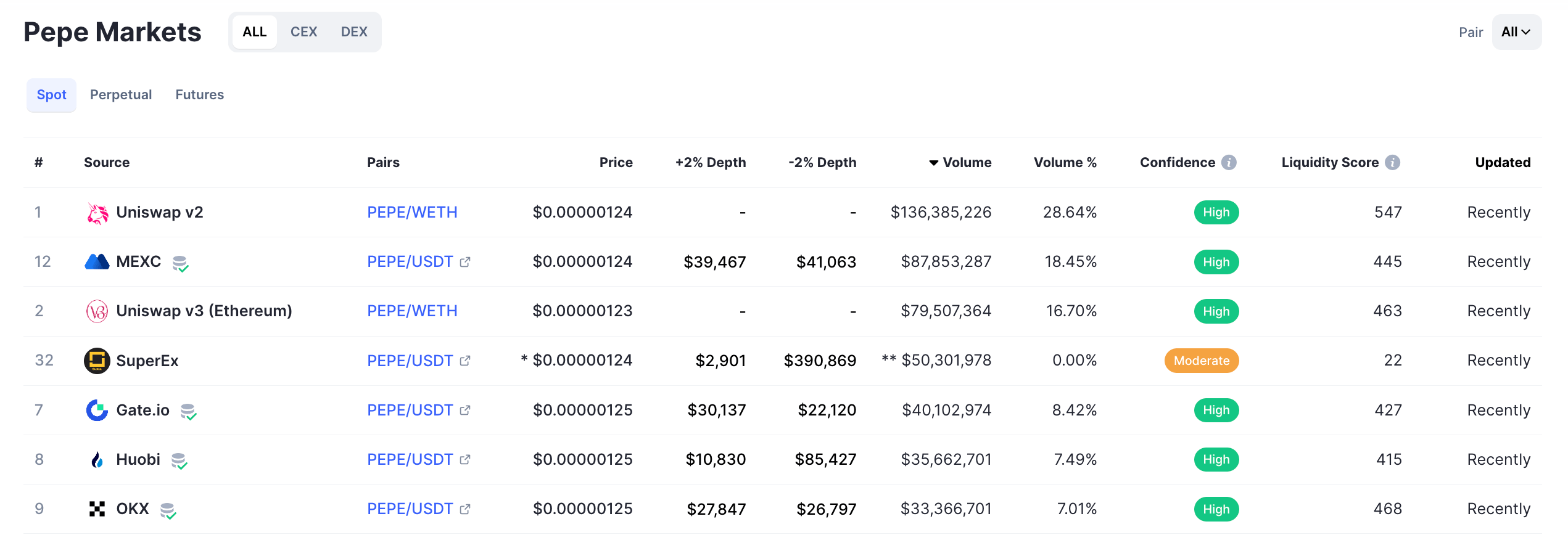This image showcases a webpage from a cryptocurrency website named "PepeMarkets." At the top-left corner, the site's name "PepeMarkets" is bolded. Adjacent to the name is a white-highlighted rectangle with the word "ALL," followed by options labeled "S-E-X" and "D-E-X."

Beneath this header, there's a blue-highlighted label "SPOT" within a gray box. Next to it are other trading options such as "Perpetuals" and "Futures." On the far right of the header, there's a section labeled "PAIR" with a drop-down arrow in a light gray box for selecting trading pairs.

The next section down features columns labeled "NUMBER," "SOURCE," "PAIRS," "PRICE," "DEBT," "VOLUME," "VOLUME PERCENTAGE," "CONFIDENCE," "LIQUIDITY SCORE," and "UPDATE." 

Following this, the table begins with:
1. "UNISWAP," detailing information about trading pairs, pricing, and volume. The confidence level is noted as high, followed by a timestamp "RECENTLY."
2. "MEXI," showcasing pairs like "PEPE/USDT," along with the price and trading details in the same format as UNISWAP.
3. Additional exchanges listed include "UNISWAP B3," "ETHEREUM," "SUPERX," "GATE.IO," "HUOBI," and "OKEX," each with information regarding pairs, prices, volume, and other relevant trading details.